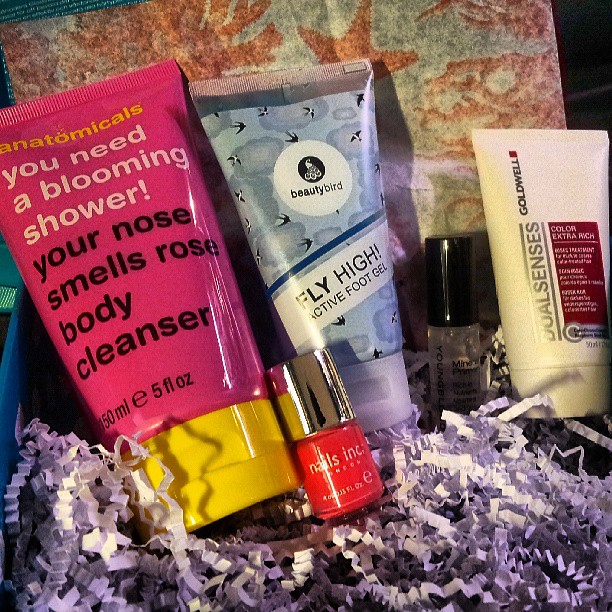The photograph features a variety of beauty and personal care items neatly arranged on a bed of wrinkled, accordion-like packing material in purple and white. On the far left, there is a pink squeeze bottle with a yellow cap labeled "Anatomicals You Need a Blooming Shower Your Nose Smells Rosy Body Cleanser," detailing it as 50ml or 1.69FL-OZ. Beside it, a small, reflective silver-capped jar showcases red nail polish branded as "Nails Inc." Moving to the right, a squeeze bottle with a blue and purple cloudy design bears a white circular label with a black bird logo and the words "Beauty Bird Fly High Active Foot Gel," finished with a purple cap. Adjacent to this bottle, there is a clear liquid in a small bottle with a black lid, resembling a spray sanitizer. Finally, on the far right, a yellow squeeze bottle is marked with "Goldwell Dualsenses Color Extra Rich," featuring an amber square on the top right corner and culminating in a white cap that touches the packing material below.